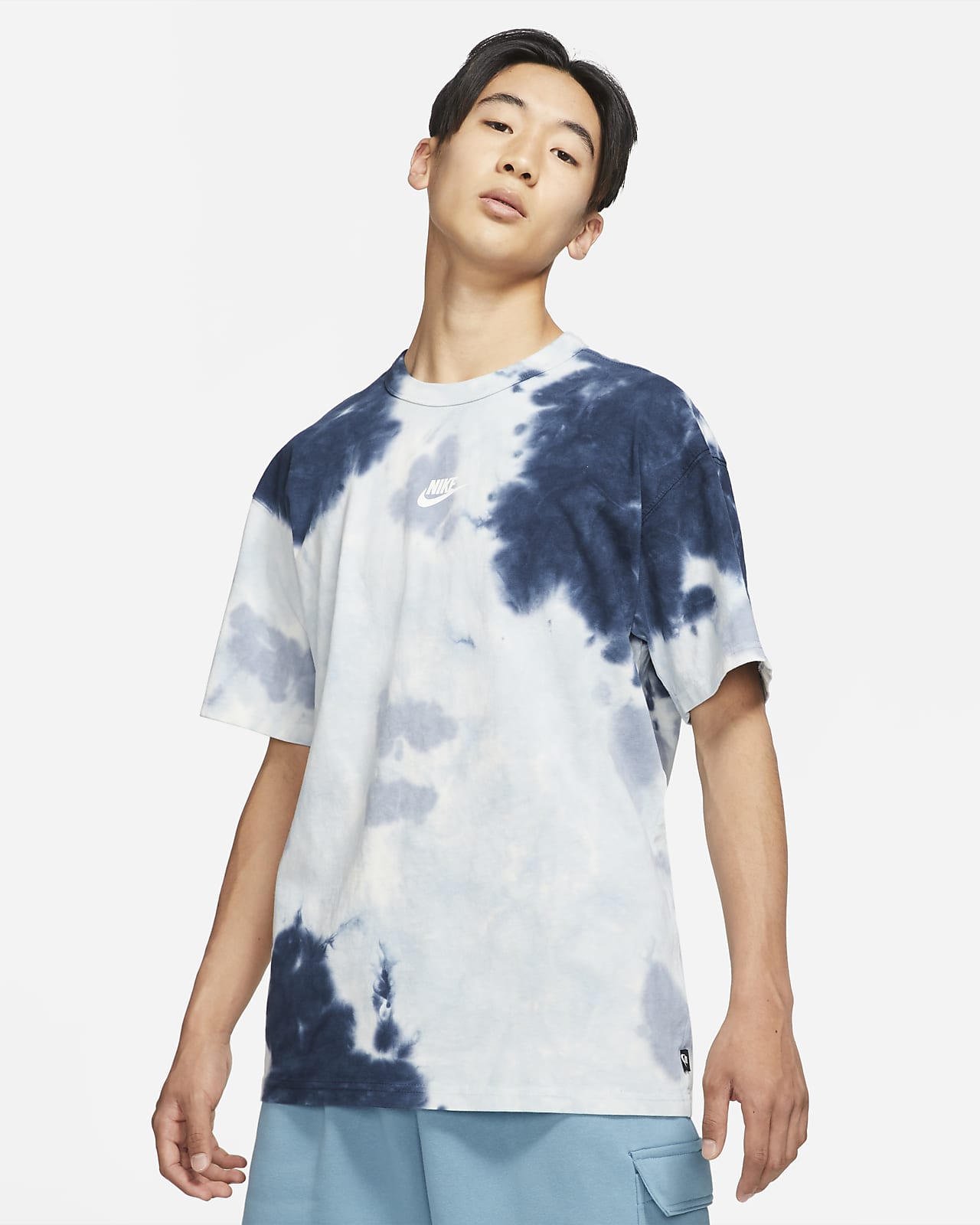The image features an Asian young man of slender build, standing confidently in front of a gray backdrop. His black hair is parted in the middle and reaches down to his ears, framing his face as he tilts his head slightly to the side. His eyes are keenly focused on the camera, giving off a sense of arrogance or self-assuredness. He is dressed in a tie-dye Nike shirt that combines shades of navy blue, light blue, and gray, prominently displaying the white Nike logo. His bright blue cargo shorts have a visible pocket on the left leg. With his hands poised near his pockets, he stands with a confident and assertive posture, positioned centrally in the frame with a balanced space above his head.